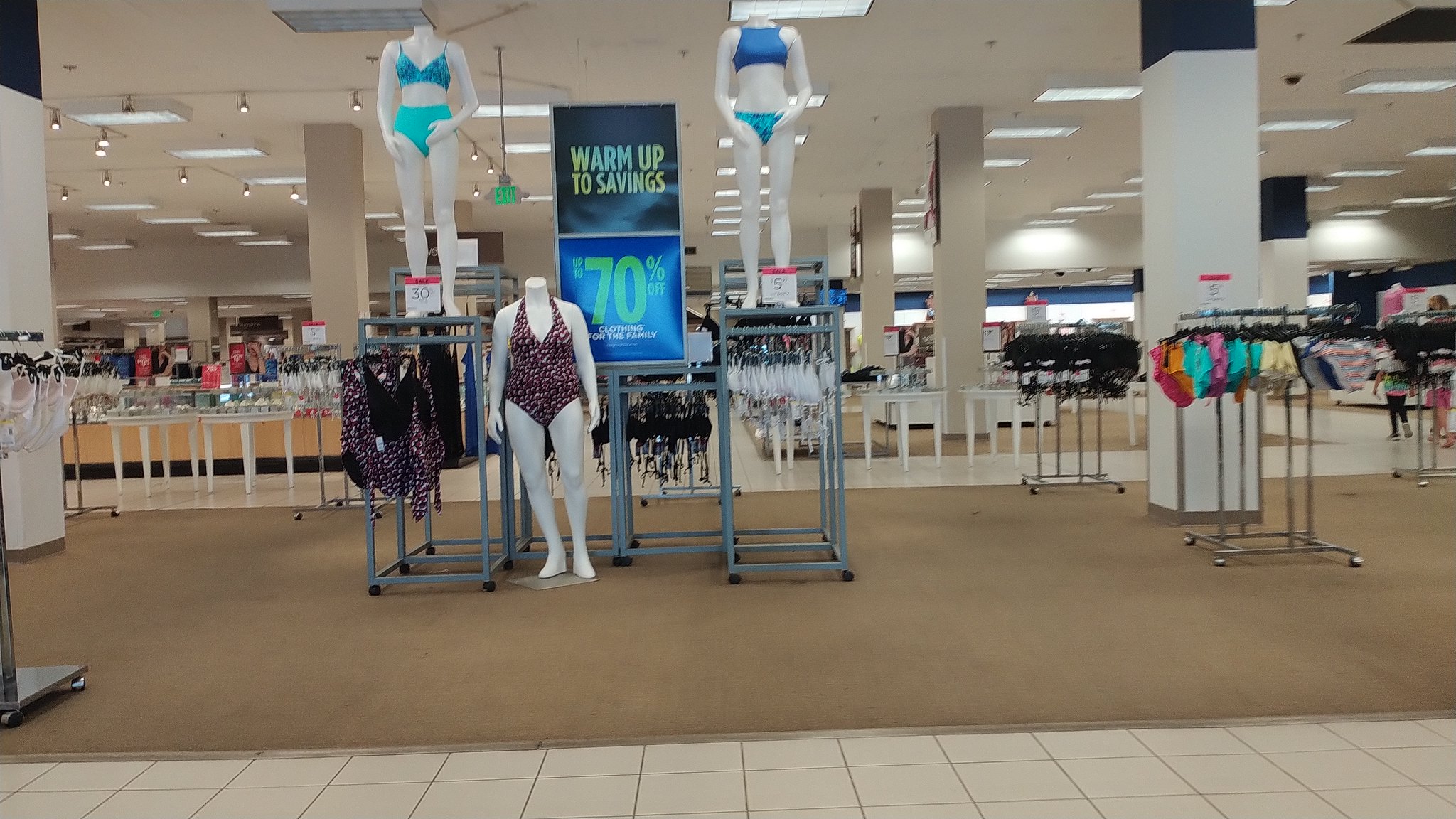This image captures the vibrant entrance of a storefront within a mall. Displayed prominently at the front are mannequins showcasing a variety of women's swimsuits, including both one-piece and two-piece designs. The display area features multiple "four-way" clothing racks adorned with various swimsuit styles and sizes, each marked with colorful sale signs. A prominent banner above reads "Warm Up to Savings, Up to 70% Off," complemented by additional signs on the racks indicating discounts like "30% Off" and various other markdowns. The store's interior, illuminated by bright lighting, reveals more of its layout. In the backdrop, a jewelry counter is visible, flanked by shoppers browsing other merchandise. The scene effectively conveys the bustling, inviting atmosphere of a mall store geared towards swimwear and summer savings.